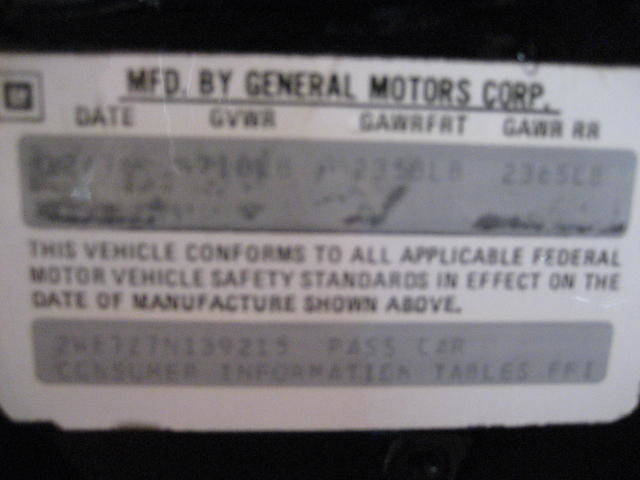The image depicts a close-up of a vehicle manufacturing plate affixed to a black background. The plate is a white sticker with black text that reads, "Manufactured by General Motors Corporation." Just below this, there’s a space for the date, though it’s difficult to read due to the photograph’s blurriness. Below the date area, the text states, "This vehicle conforms to all applicable Federal Motor Vehicle Safety Standards in effect on the date of manufacture shown above." Further down, more detailed information includes the label "2WE727N139215PASSC&R Consumer Information Tables FFI," indicating the vehicle’s VIN number and that it’s a passenger car. The repeated emphasis on compliance with safety standards and vehicle identification underscores the plate’s importance for regulatory and informational purposes.